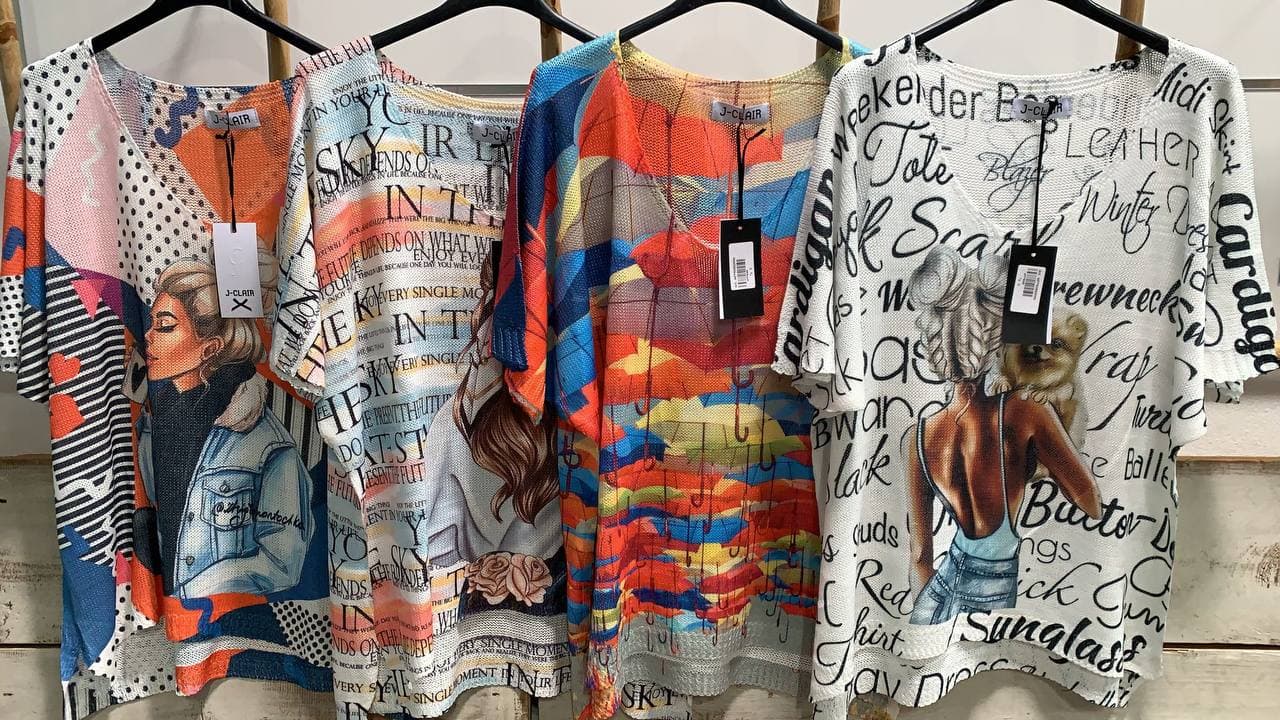This image showcases four women's boho tunic style t-shirts with scoop necks and short sleeves, artfully displayed on black hangers against a whitewashed reclaimed wood wall. The shirts feature a variety of vibrant colors and graphic designs, each with distinct and detailed artwork. 

From left to right:
1. The first t-shirt is predominantly black and white, highlighting a graphic of a girl holding a Pomeranian. 
2. The second shirt is adorned with multi-color umbrellas stacked on top of each other, creating a playful and lively visual.
3. The third shirt, partially obscured, displays topographical patterns interspersed with colors like orange, red, blue, green, and yellow. A girl features among the design elements.
4. The fourth and rightmost shirt presents black-colored text against a white background. Words such as "winter," "toad," and "scary" are scattered around a central image of a girl in a backless gown, her hair tightly pulled back, with a dog draped over her shoulder.

Each t-shirt bears visible tags indicating the brand, which appears to be "J.Claire" (J-C-L-A-I-R). The hangers are cut off at the top, slightly cropped out of view. This carefully arranged display hints at a stylish garment shop's interior, providing a visually appealing and colorful clothing selection.